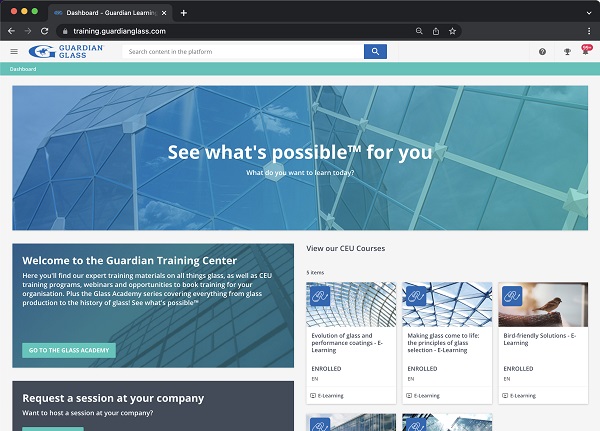An image of the Guardian Glass Training Center website is depicted. The website URL, training.guardianglass.com, is visible in the browser’s address bar, confirming the site. The top browser header is black, featuring the standard red, yellow, and green stoplight-style buttons for window management.

In the website header, the Guardian Glass logo, a stylized 'G' in blue, is prominently displayed. The header itself is a bluish-aqua color, creating a modern and professional look.

The central focus of the webpage is a large image accompanied by the text "See what's possible for you." The image showcases a futuristic, glass-structured outdoor garden dome, evoking a sleek and innovative atmosphere. Beneath this visual, a welcoming message reads: "Welcome to the Guardian Training Center. Here you'll find our expert training materials on all things glass as well as CEU training programs, webinars, and opportunities to book training for your organization, plus the Glass Academy series covering everything from glass production to the history. See what's possible. Go to the Glass Academy."

Additional sections on the page highlight various CEU courses available for enrollment, including "Evolution of Glass," "Making Glass Come to Life: The Principles," and "Berg Friendly Solutions Learning." Each course is labeled as enrolled. There is also an accessible button to "Request a Session at Your Company," although the lower part of the webpage where this appears is incomplete in the caption provided.